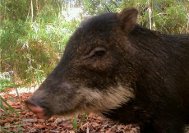This small photograph features a close-up head and neck shot of what appears to be a wild boar or warthog, facing towards the left. The animal's fur is mostly dark brown with black accents, but it has distinctive white and beige fur under its chin and neck. Its snout is long and flat, with a flesh-colored tip at the nostril. The rounded ears and black eyes add to its characteristic facial features. The background is a mixture of blurred trees at a distance and a ground strewn with dark brown leaves and patches of grass. The image also captures a sliver of light blue sky at the top. The rocky and possibly creek-laden terrain at the bottom of the photograph hints at a diverse natural habitat.